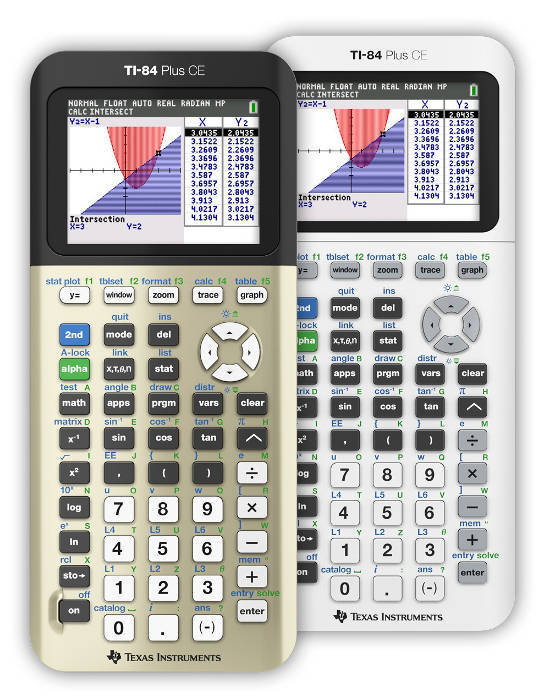This image features a professional-looking photograph of two advanced scientific calculators by Texas Instruments, specifically the TI-84 Plus CE models. The calculators are positioned with one slightly stacked atop the other on a flat surface. The calculator on the left has a sleek design with a black frame around the screen, and its body transitions from a darker top to a light silver bottom. It features several multi-colored buttons, including some white and gray ones, with specific keys marked "Window," "Zoom," "Trace," and "Graph," along with directional arrow buttons. 

The calculator on the right is primarily white and sports a prominent black frame around its activated screen, which displays various operational states: "normal," "float," "auto," "real," "radian," "MP," and "intersect." Notably, a green battery indicator shows a full charge. Both calculators have a distinctive and professional appearance, ideal for complex mathematical tasks such as graph plotting and formula computation. The color scheme of the buttons includes blue, green, black, and white, designed to differentiate functionality and enhance usability. Overall, the image effectively showcases these slender, flat devices, highlighting their extensive capabilities and sleek design.